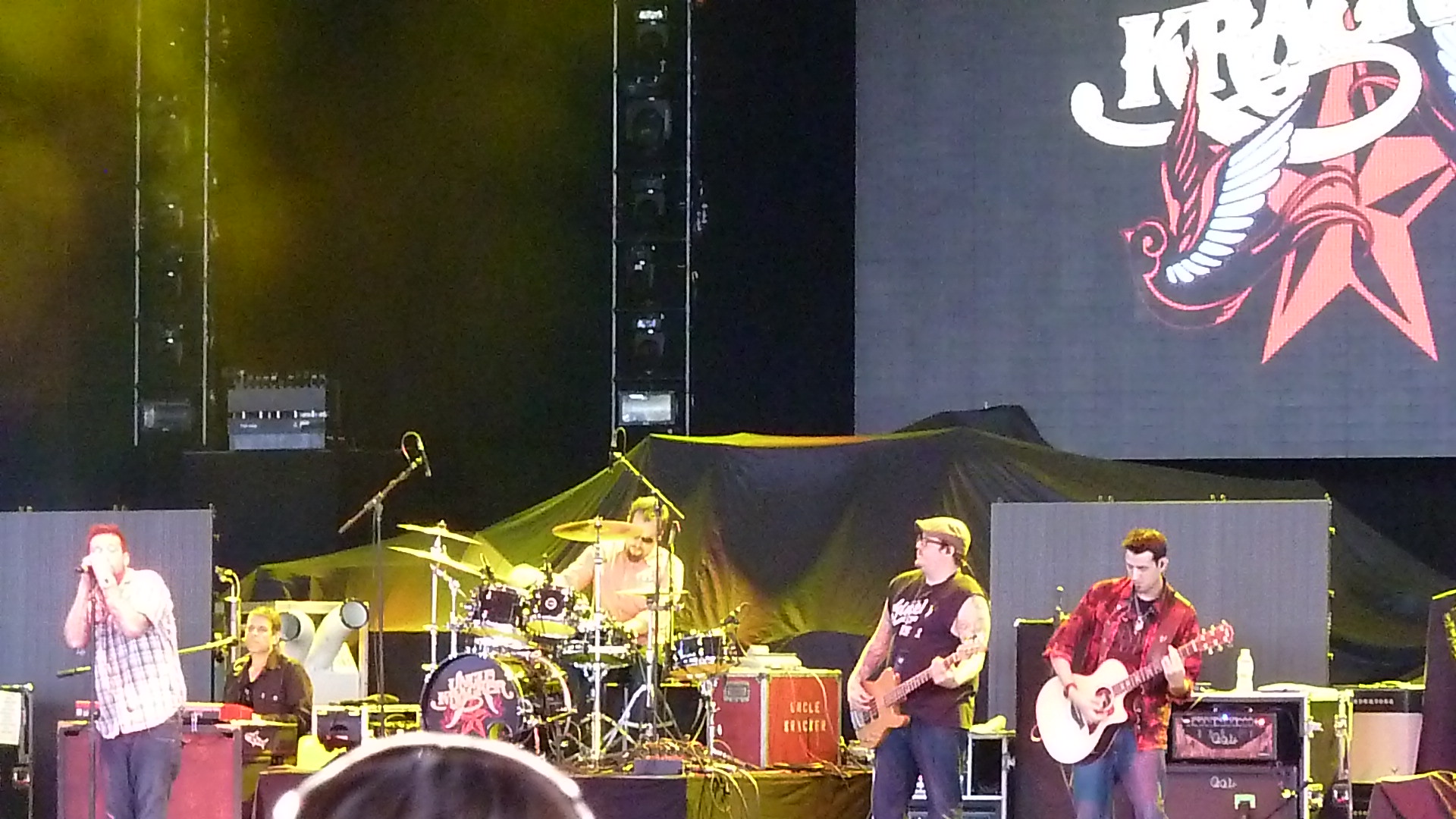The image captures an energetic concert scene featuring the band Uncle Kracker. The stage is illuminated with yellow light, highlighting the musicians as they perform in front of a large, vividly decorated screen. The screen showcases the band's logo, which includes white text, a pinkish star, and an illustrated bird with pink and white wings. On stage, the lineup includes two guitarists positioned on the right, a drummer in the middle, a keyboardist to the left, and the lead singer standing at the front. Amplifiers and a large black tarp are visible behind the performers, suggesting a well-equipped setup. Additionally, the drum set and one of the red amplifiers have "Uncle Kracker" emblazoned on them, cementing the band's identity. The photo appears to be taken from within the crowd, as a partial view of an audience member’s head slightly obscures the drum set, emphasizing the live concert ambiance with giant walls of speakers surrounding the stage.